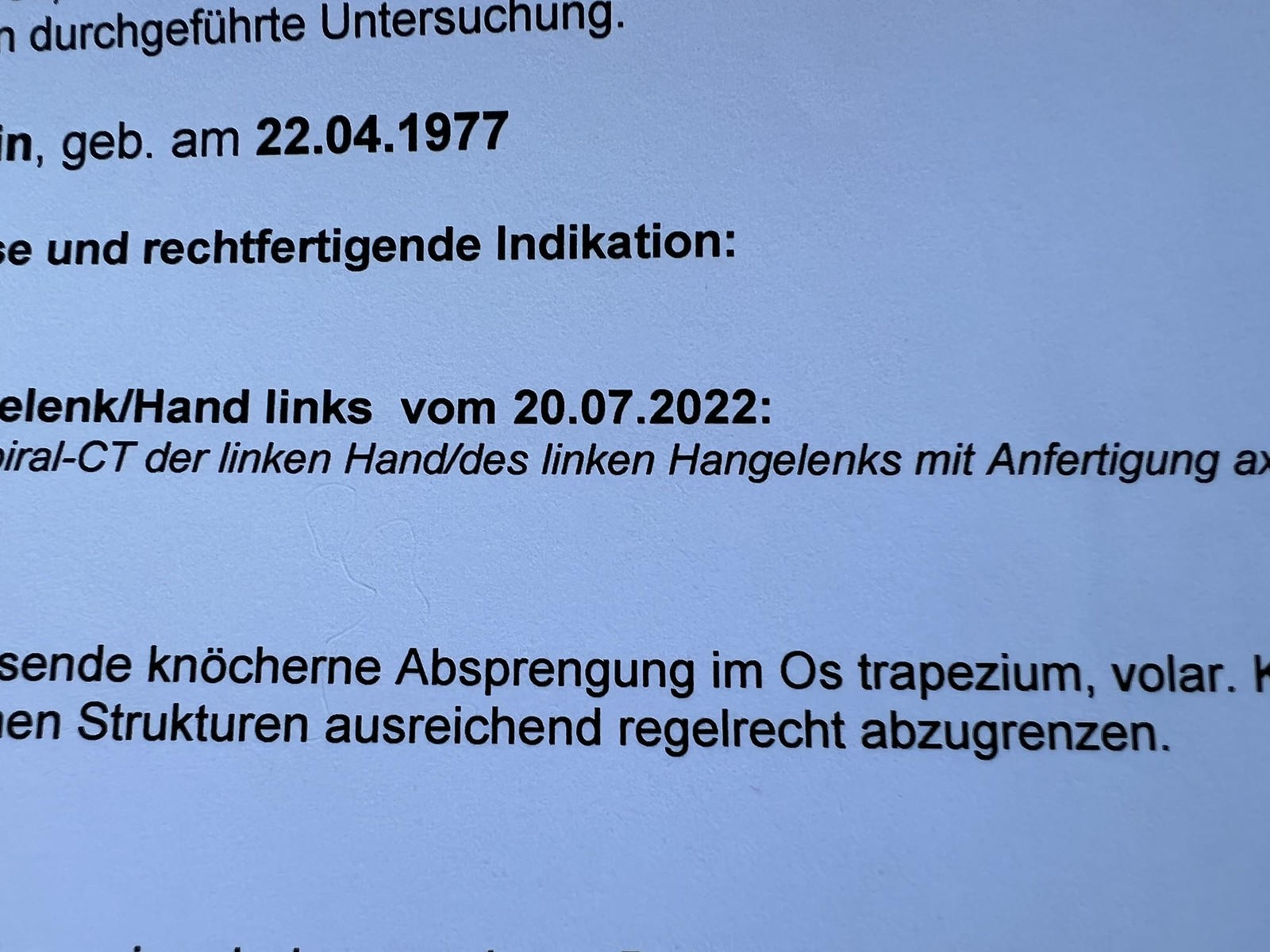The image displays a piece of paper, possibly an official record or poster, featuring multiple lines of German text on a light blue background. The text is predominantly in sans serif font, with some parts bolded for emphasis while other sections are italicized. The sentences are in black, with some sections in bold black text. The upper left section features the words "DURCHGEFUHRTE" and "UNTERSUCHUNG." Directly beneath are dates: "22.04.1977" and "20.07.2022," with the latter positioned centrally in the image. Additional lines of text appear below these dates, ending with the words: "Strunk Turin," "Ausrachend," "Regelrecht," and "Absurgerenzen." The image captures a blend of numbers and words, some of which are cropped off at the edges, adding to the official yet slightly obscured nature of the document.